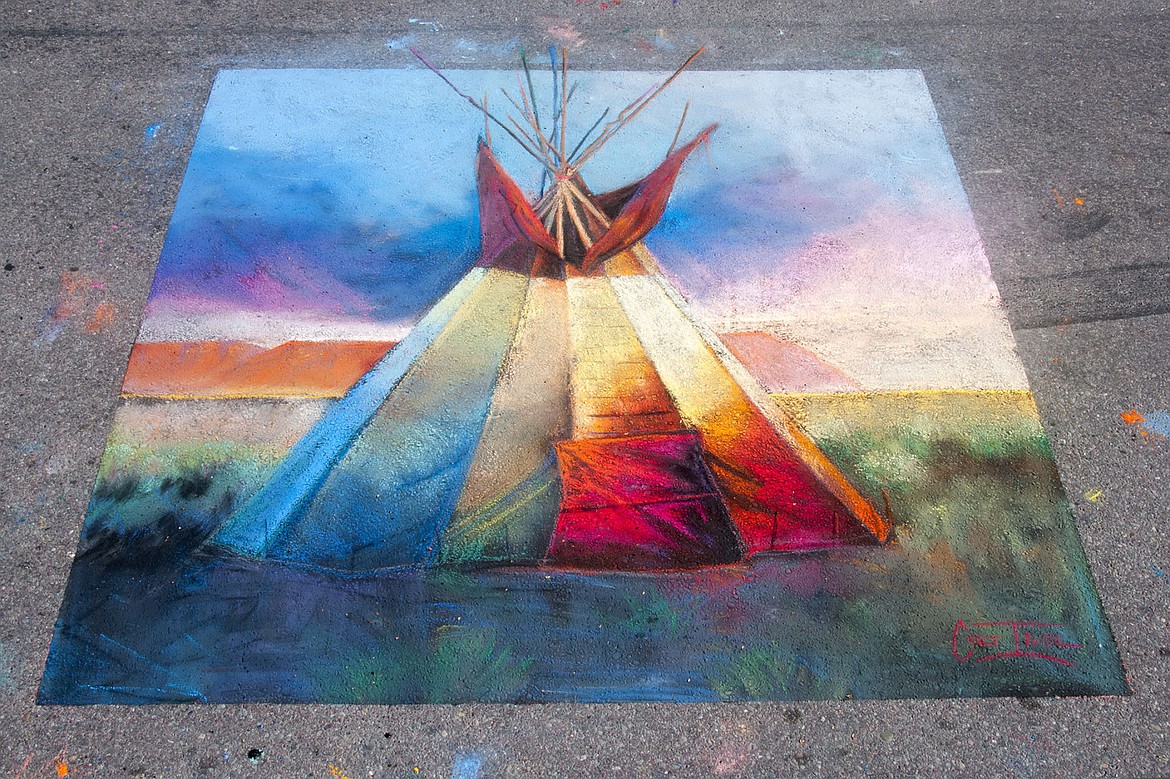The image depicts a vibrant and detailed chalk drawing on a piece of concrete, resembling a painting. Central to the artwork is a colorful teepee, triangular in shape, with pieces of wood protruding from its top, which is adorned with an orangish-red hue. The teepee features various panels: two bluish, one beige with a hint of green, another beige with red at the bottom and a square detail, and two reddish-orange. This structure is set against a sky painted in shades of blue, white, and pink, evoking a cotton candy appearance. Behind the teepee, there’s an orange, mountain-like region, suggesting a picturesque landscape. At the base of the teepee is bluish-green grass, adding to the natural setting. The entire artwork rests on a light gray, asphalt-like concrete surface. In the bottom right corner, there appears to be an artist’s signature in red, though it is somewhat illegible.